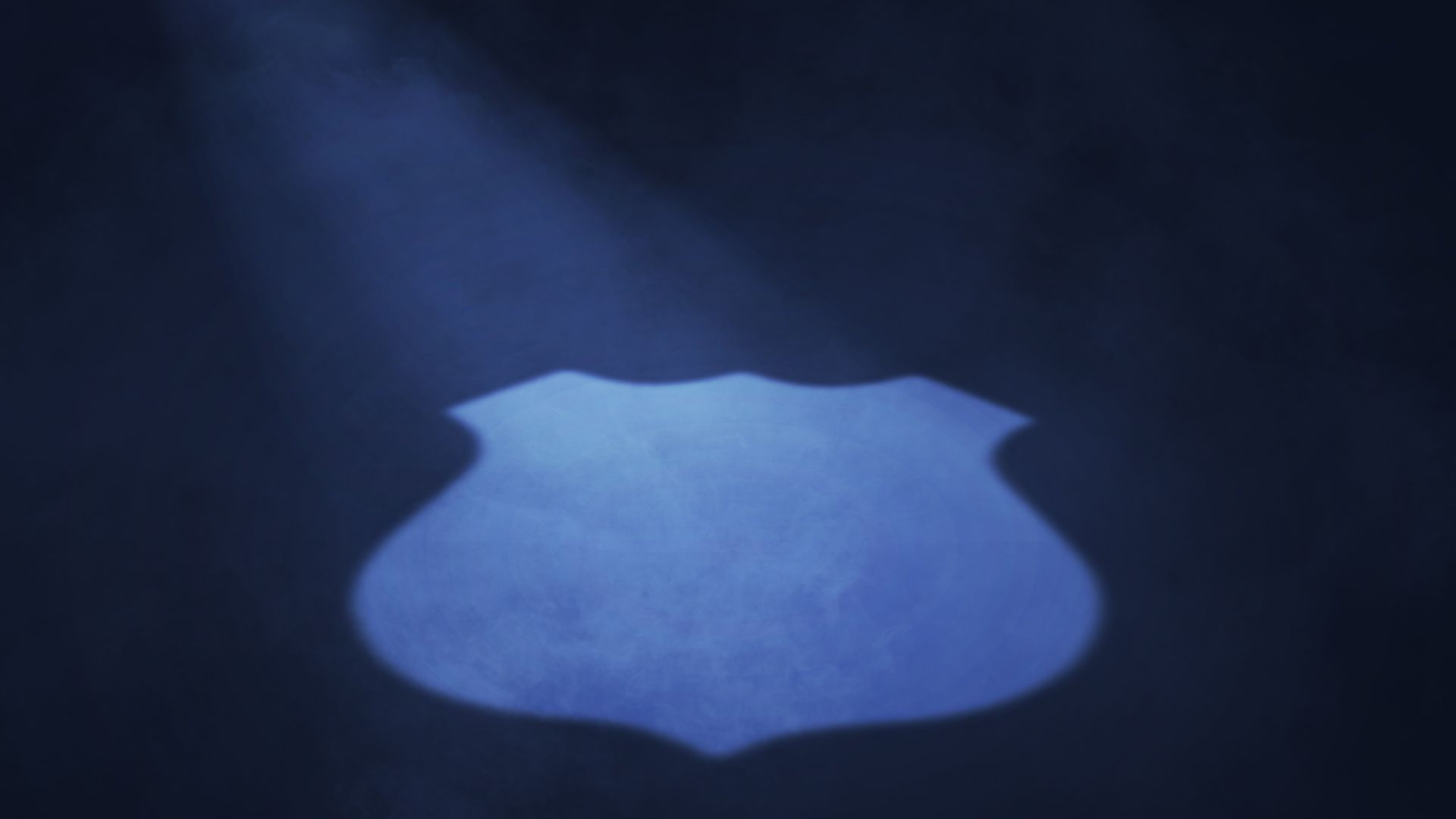The image features a striking dark black background, accentuated by a single prominent shape in the center towards the bottom. This shape closely resembles the form of a police badge or shield, characterized by its light blue color and jagged edges at the top, tapering down to a point at the bottom. The shield shape appears thick and three-dimensional against the stark, contrasting backdrop. Additionally, there is a distinct bluish streak that runs through the upper part of the image, directly above the shield, further highlighting its presence. The overall composition suggests that the shield is being illuminated, creating a spotlight effect that emphasizes its form in the darkness.